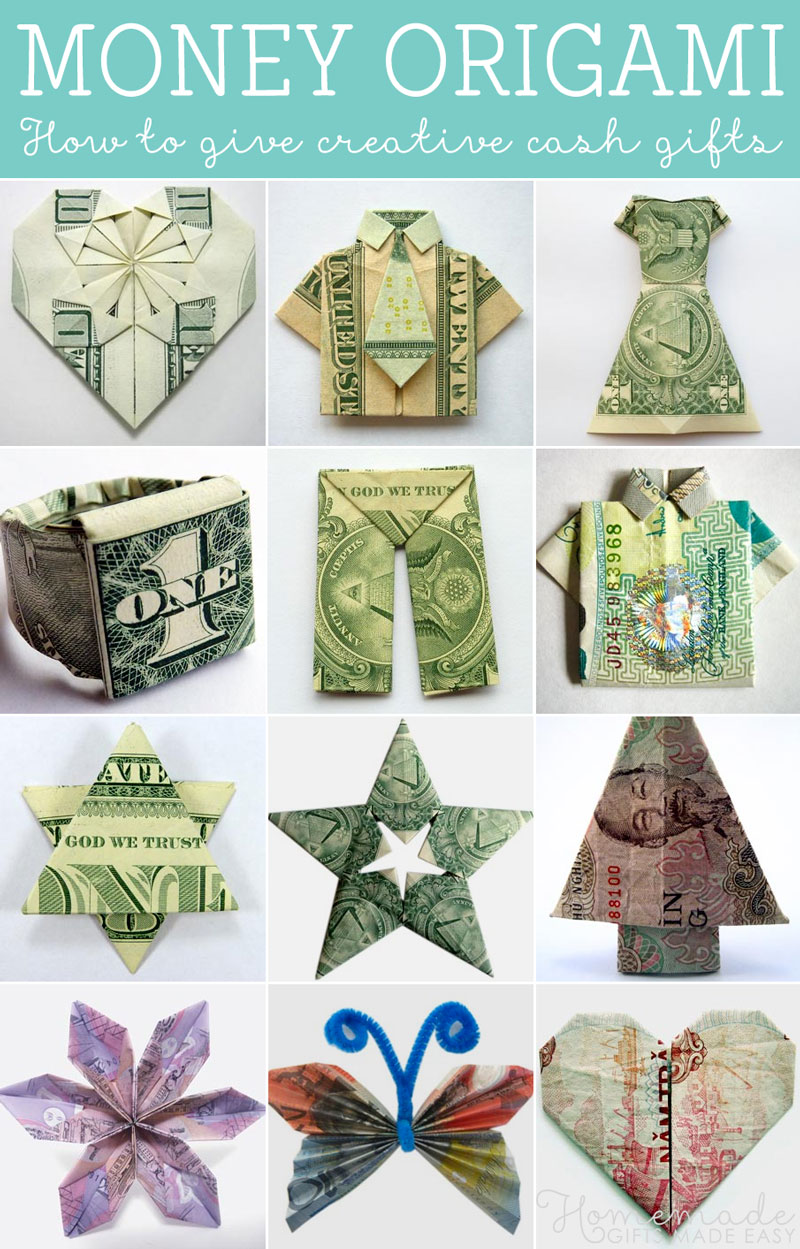The image is a vertically structured poster featuring a thick green border at the top with the heading "MONEY ORIGAMI" in bold white letters and underneath, in cursive writing, it reads "How to Give Creative Cash Gifts." Below this are four rows of images, each consisting of three photographs showcasing various origami objects crafted from currency. 

In the first row, the leftmost image shows a $10 bill folded into a heart. To its right, there is a $20 bill shaped into a shirt complete with a tie, followed by a $1 bill transformed into a dress. The second row displays a $1 bill folded into a ring, another $1 bill made into a pair of pants, and a different bill shaped into a tree. In the third row, there's an origami star, another star featuring a star motif, and a structure resembling a snowflake or a flower. The bottom row includes international currency folded into objects like stars, butterflies with distinct red-and-blue wings, and a heart, possibly made from a Chinese bill. Each row's images are uniformly sized, emphasizing the intricate details and creativity of the money origami.